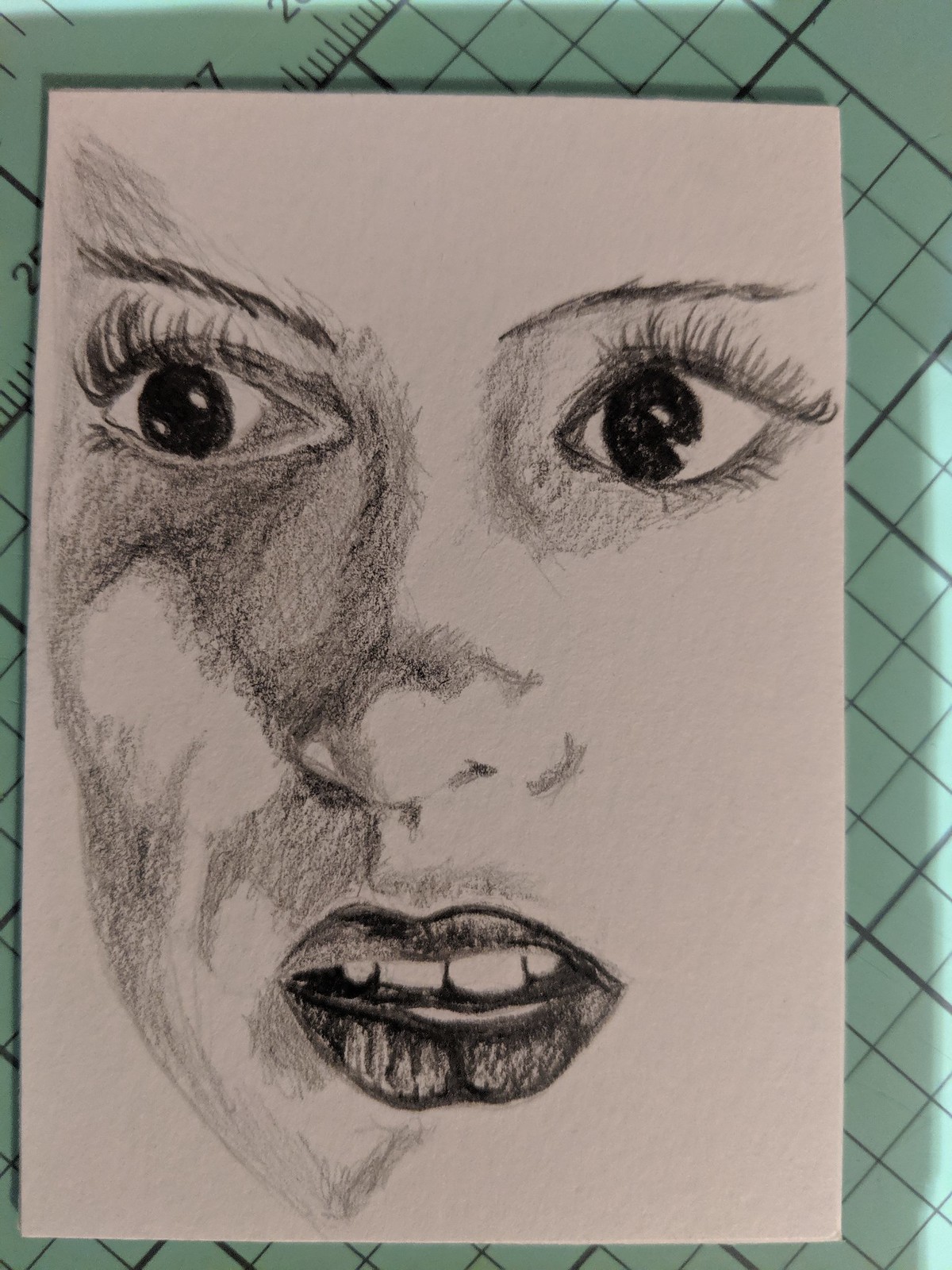A detailed pencil drawing captures a close-up of a woman's face, rendered on a green graph paper background. The drawing showcases an intricate crosshatching technique to depict shadows and textures. The woman’s expression is one of alarm; her wide eyes and slightly open mouth reveal a sense of sudden surprise, as if she has encountered something unexpected and unsettling. The drawing focuses solely on her face, omitting her hair and ears, directing all attention to her vivid, startled eyes and the tension in her parted lips that subtly reveal her teeth. The meticulous crosshatching enhances the depth and intensity of her expression, making her emotions strikingly palpable.